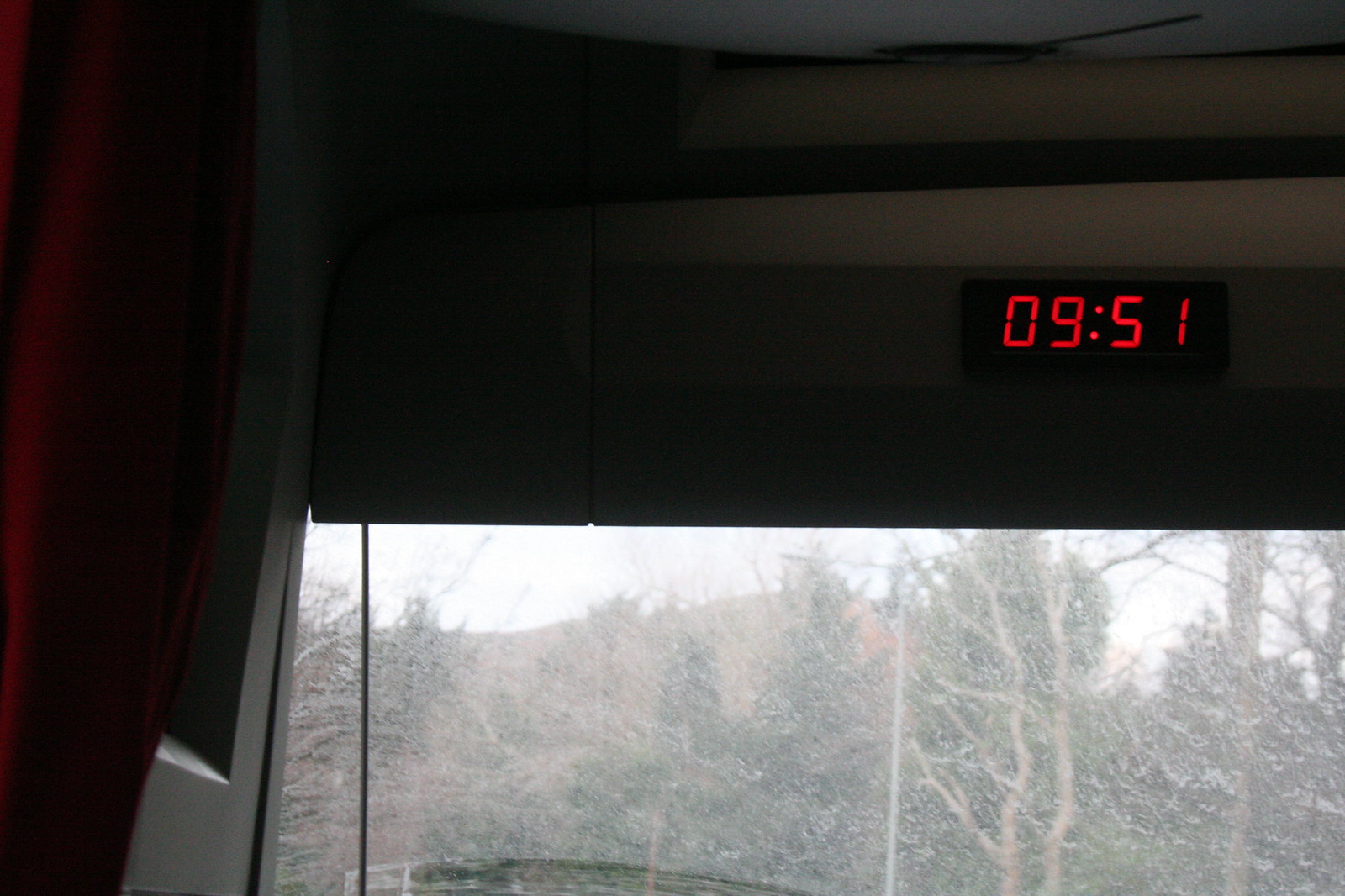A rectangular window from the interior of a building or vehicle frames a wintry landscape. Heavy snowfall obscures much of the view, creating a serene yet almost ghostly ambiance. Barely visible through the thick snowflakes, the tops of snow-covered trees stand against the backdrop of a distant mountain. The weather appears harsh and extremely cold. In the upper right-hand corner of the scene, a digital timer or clock displays "09:51," which could indicate either the time—9:51 AM—or a countdown of 9 minutes and 51 seconds. Despite the daylight, the storm renders the visibility quite poor, casting an ethereal blanket of white over the entire landscape.